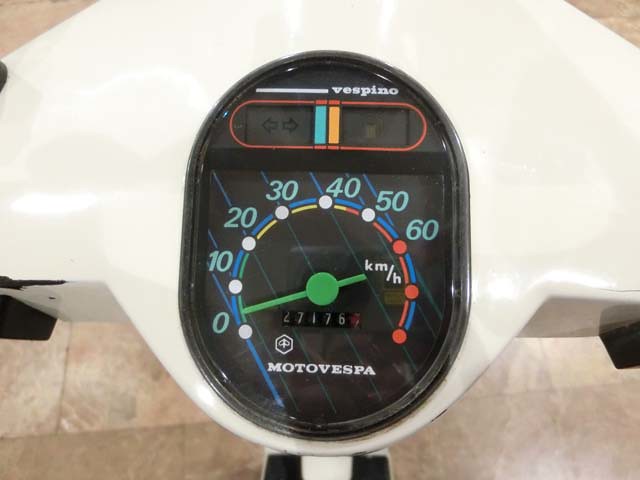The image showcases a top-down view of a vintage Vespa scooter's dashboard, highlighting its intricate details. The dashboard is set within a white metallic or plastic surface, reminiscent of an airplane wing, while a cream-colored tiled floor is visible in the background.

At the forefront, there is a large, black, oval dial with a white bar at the top that reads "Vespino." Below this, a smaller rectangular gauge houses turn signal indicators and a faded gas gauge that are not lit up. The primary dial is a speedometer marked in kilometers per hour (km/h), featuring a green needle. The speedometer face is labeled "Moto Vespa" in white text.

The speedometer dial includes a distinctive blue circle, a green arc indicating speeds between 0 and 20 km/h, a yellow arc between 20 and 45 km/h, and a red line from 45 km/h upwards, emphasizing caution or maximum speed. This detailed portrayal captures the classic design and functionality of the vintage Vespa scooter.